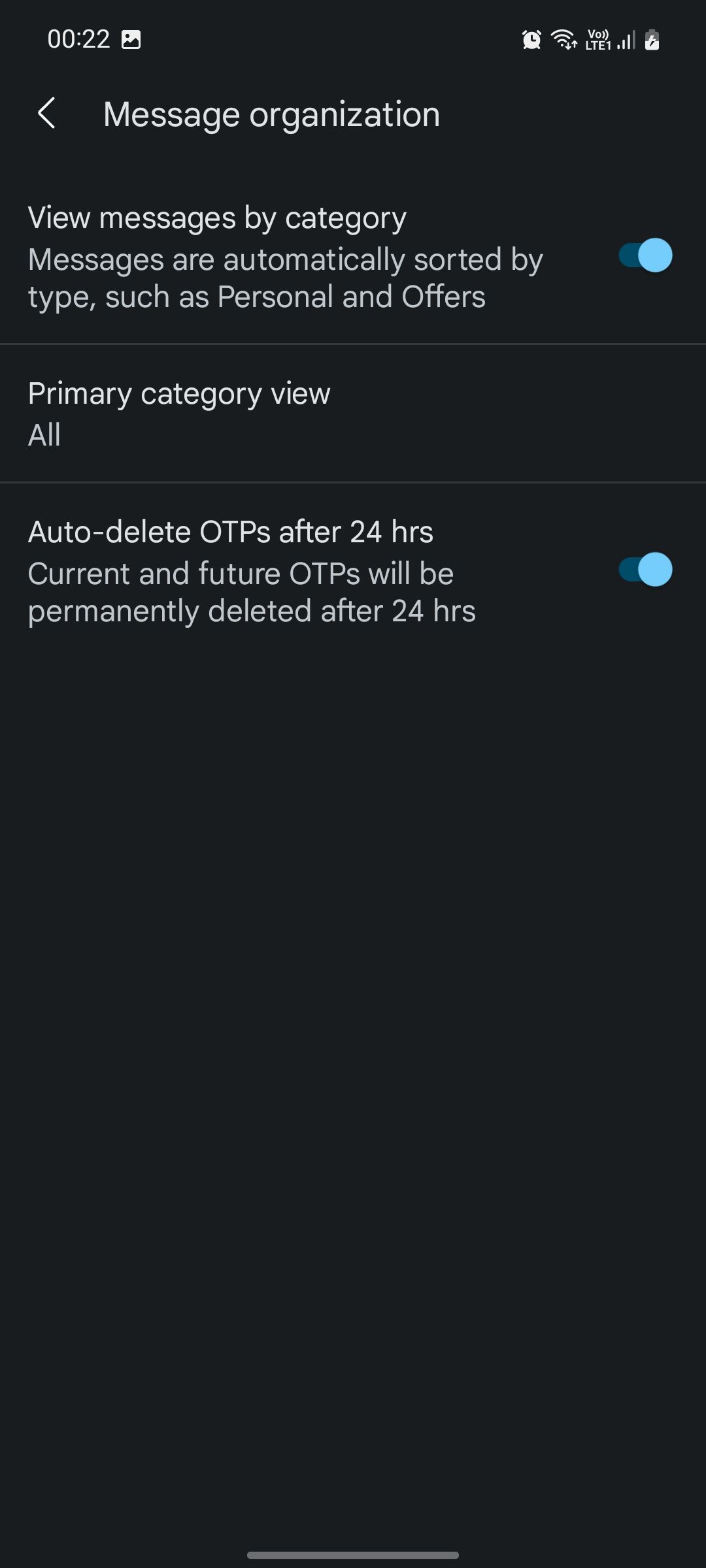A screenshot displaying a cell phone's settings page is featured. Indicators in the upper right corner confirm it is a cell phone, with a battery icon, signal strength bars, and a 4G/5G connection symbol visible. The upper left-hand corner shows the time in a 24-hour format, commonly known as military time, which is less familiar to American users.

Dominating the center of the screen is a section titled "Message Organization," suggesting the user has navigated into their settings to adjust how incoming messages are sorted and handled. The interface is stark, with a black background contrasted by white text and various light blue toggle switches. These toggles allow the user to enable or disable specific features related to message management. Three distinct message organization options are present, each with active toggles, indicating the user has enabled all available settings for optimal message organization.

The design and chosen settings imply that the user has prioritized thorough and organized handling of incoming messages.